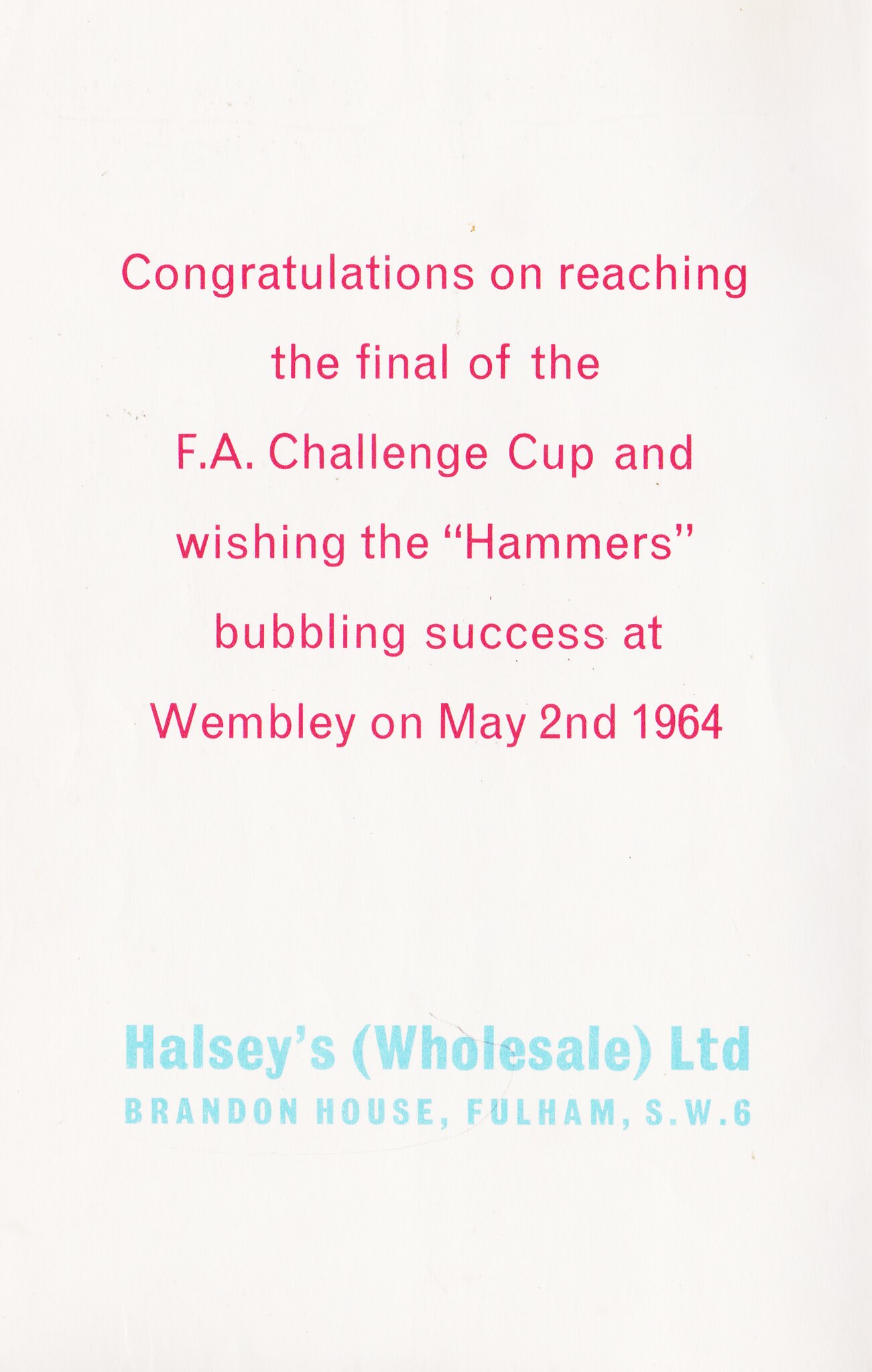The image is a vertical-oriented page resembling a vintage flyer or magazine excerpt with an off-white, textured background and some distress marks. Center-aligned, the primary section of text is a congratulatory message rendered in six lines of pink font: "Congratulations on reaching the final of the FA Challenge Cup and wishing the Hammers 'bubbling' success at Wembley on May 2nd, 1964." Below, two lines of bold blue text in a different font state the source: "Halsey's (Wholesale) LTD, Brandon House, Fulham, SW6." The text arrangement leaves a noticeable gap resembling a paragraph's spacing between the congratulatory message and the company details, suggesting it is an advertisement in support of a favored football team.